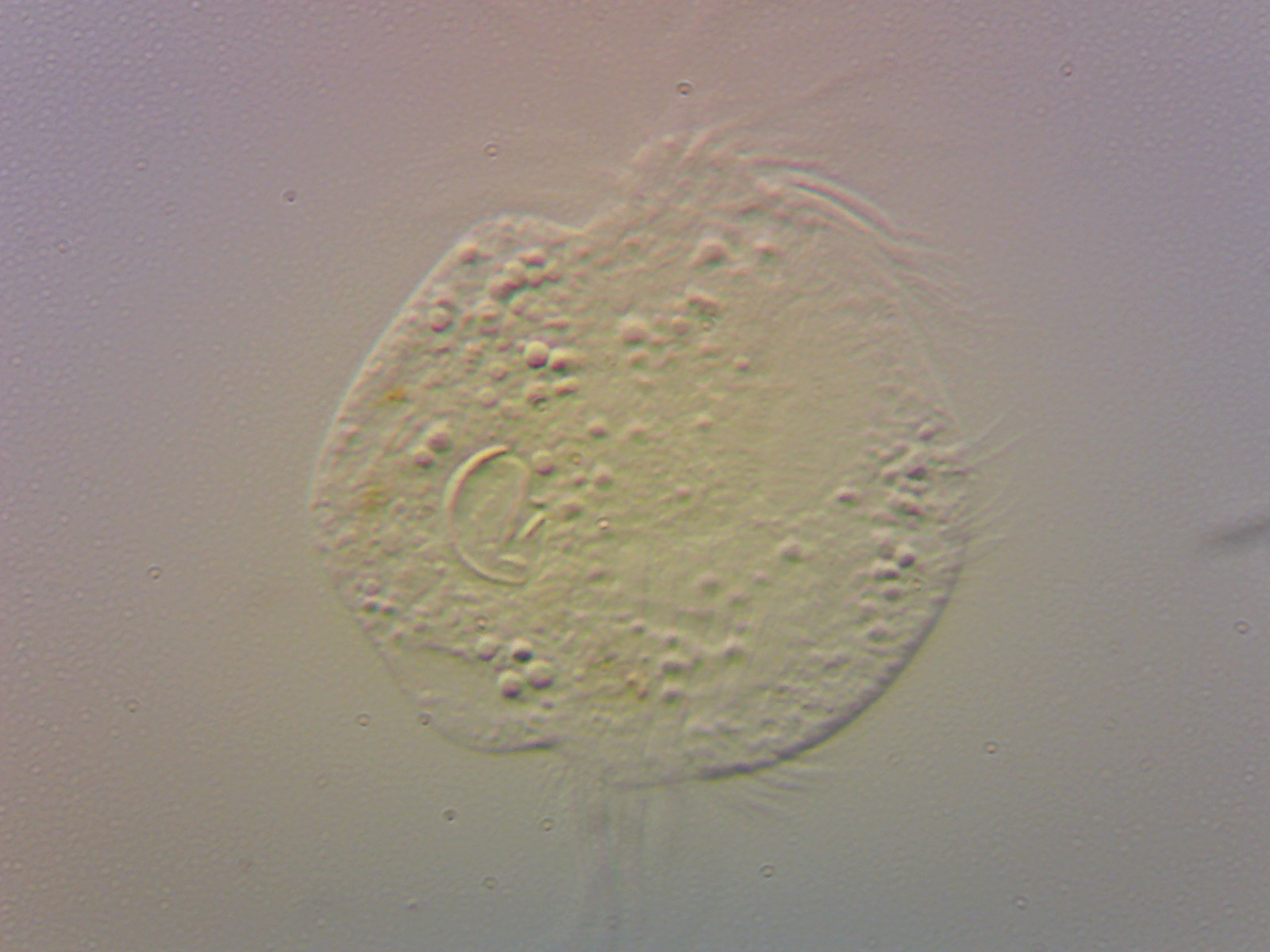This microscopic image presents a striking view of a semi-transparent microorganism, possibly a bacterium or amoeba, centrally positioned against a gradated background. The organism exhibits a rounded, lumpy shape, adorned with numerous protrusions and fine, hair-like strands extending from its body. The coloration of the core entity varies, displaying hints of green and yellow, potentially due to light reflection. The overall scene suggests it is suspended in a droplet of water, evidenced by the presence of numerous small, round particles floating around it. The background transitions from a lighter gray on the edges to an even paler shade towards the center, featuring a subtle pinkish hue at the top. The image also has an uneven texture reminiscent of ceramic bubbles interspersed with splashes of white and pink, further enhancing its intricate detail.